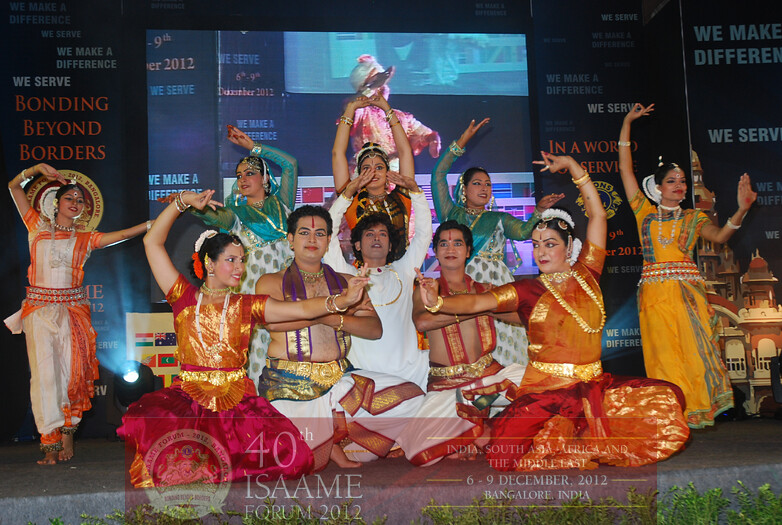This vibrant image captures the 40th ISAMI Forum 2012, held from December 6th to 9th in Bangalore, India. The event is a grand cultural performance showcasing Indian traditions. The stage is adorned with a large sign, featuring a prominent jumbotron screen and phrases such as "We make a difference," "We serve," and "Bonding Beyond Borders." In the foreground, three male dancers, dressed in colorful attire with purple, red, and green pants adorned with gold designs, are seated in the lotus position. Flanking them are two women in pink and gold saris, adorned with intricate jewelry including forehead jewels, earrings, multiple bracelets, gold necklaces, and crowns. The center of the group features a gentleman dressed in all white with a gold chain. Behind them, women in vibrant and varied dresses, such as green and orange saris, perform traditional dances with their hands and feet elegantly positioned. Their hair is tied up with bands, and some have arm decorations and elaborate gold crowns, reflecting the rich cultural heritage of India. The backdrop enhances the grandeur of the event, ensuring the essence and splendor of the Indian cultural display are vividly captured.